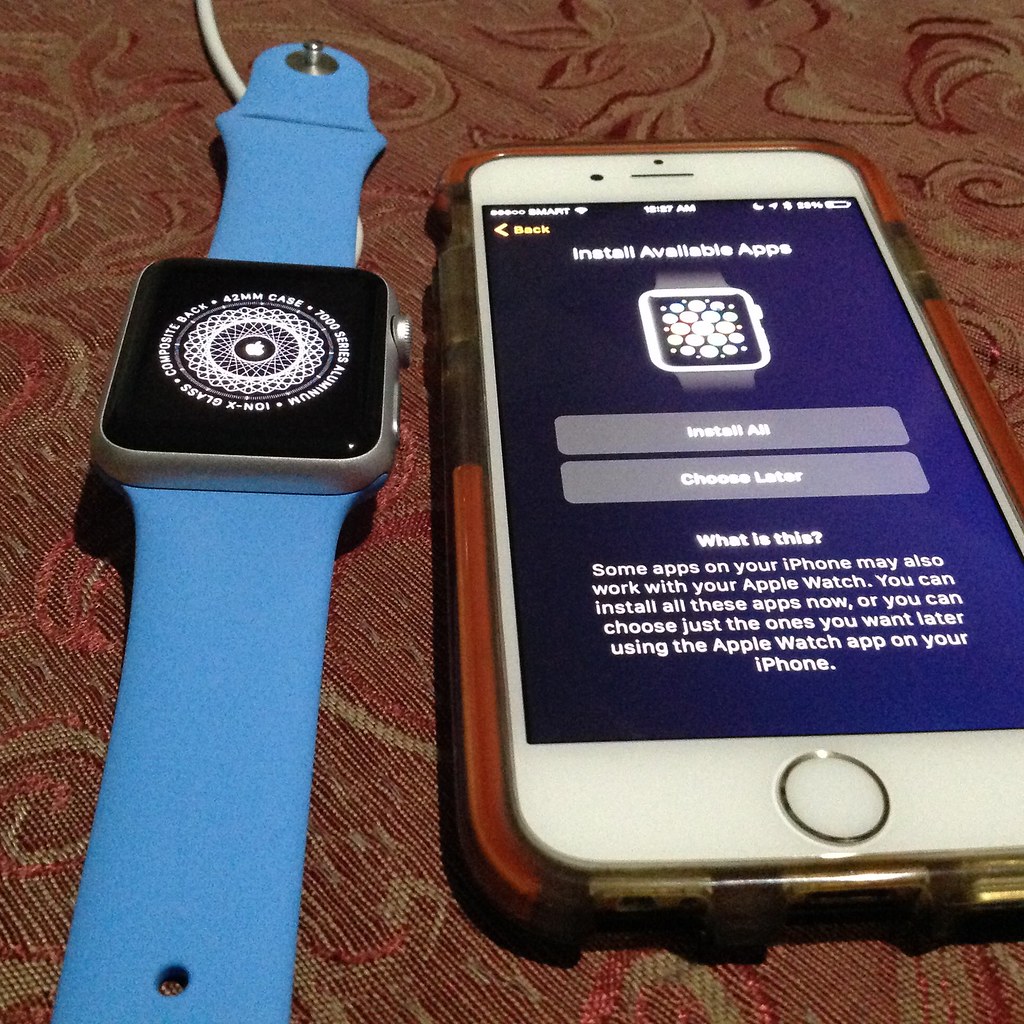The photograph features an iPhone and an Apple Watch placed on a richly colored, floral-patterned fabric that appears to be red with gold and wine tones. The Apple Watch, distinguishable by its blue wristband and the circular Apple logo sticker on its face, sits to the left. The iPhone, an older model with a home button, is on the right, displaying a setup screen for the Apple Watch. The screen message offers options to install available apps with choices "Install All" or "Choose Later." The text further explains that some iPhone apps may also work with the Apple Watch, allowing for immediate or selective installation through the Apple Watch app. This precise, technology-oriented image emphasizes the process of syncing the devices amid a warm, textured background.